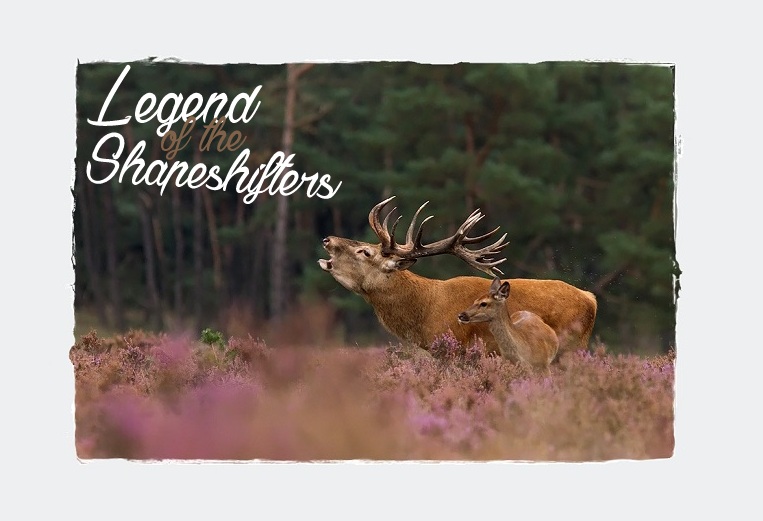This poster, derived from a color photograph, captures a serene daytime scene in nature. The image centers on a majestic male elk with a stunning rack of antlers, its mouth open as if calling out. A smaller, quiet baby elk stands next to it. Both animals are positioned sideways in a lush, blooming clover field. The background features densely packed trees, possibly coniferous, with blurred foliage adding depth to the scene. The photograph is artistically framed with a jagged, torn-edge effect and is superimposed on a light blue rectangular background. In the top left corner, in an elegant cursive script, the text reads "Legend of the Shapeshifters," with "Legend" and "Shapeshifters" emphasized and "of the" nestled between them. The stylized text and the detailed portrayal of the elk suggest influences from indigenous and Americana art, hinting at a possible use in tourism or as a vintage book cover.